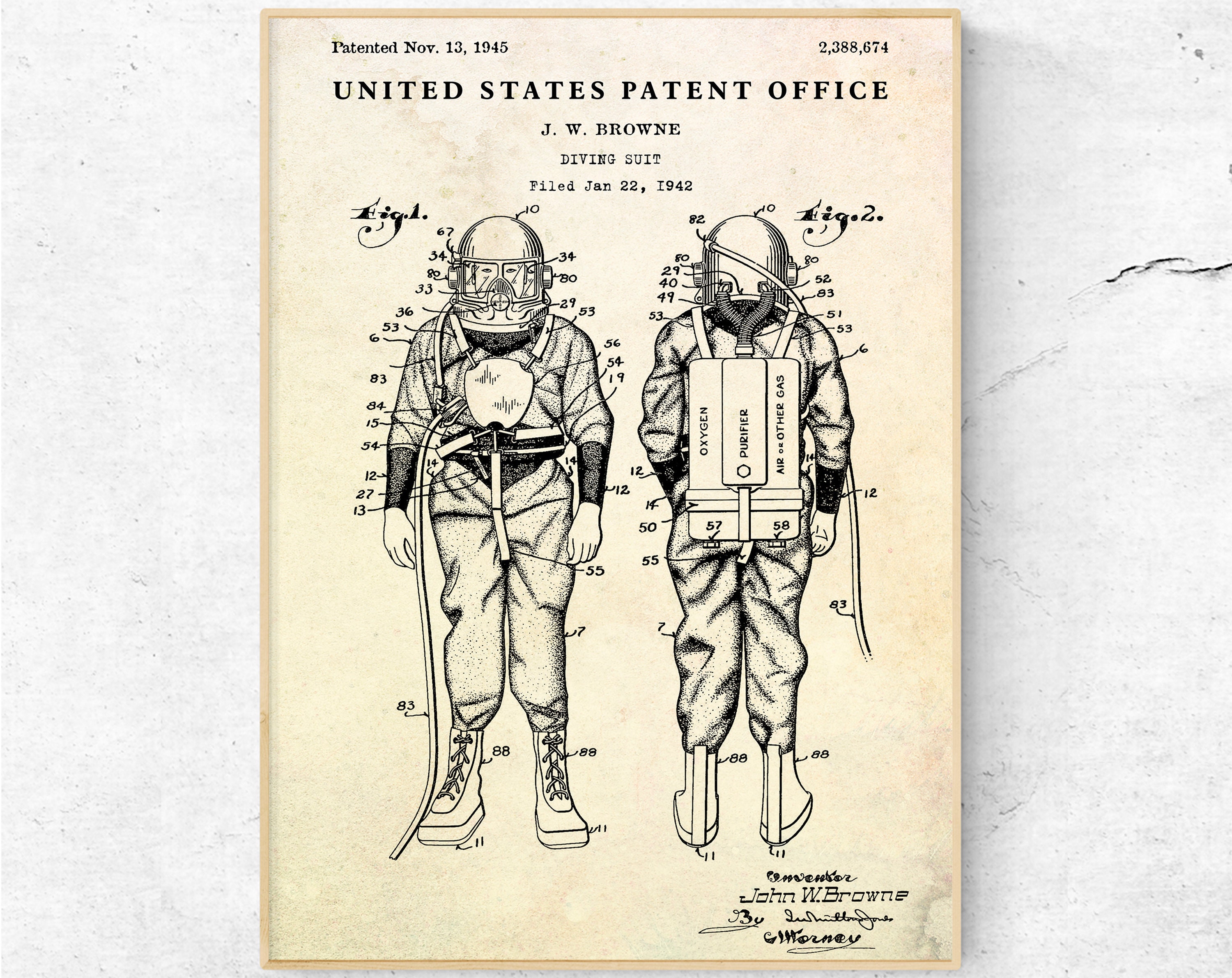This image is a historical patent diagram of a diving suit designed by J.W. Brown. The rectangular image is wider than it is tall, featuring a gray background with black lines on the right side, giving it a worn, possibly ripped effect. The central part of the image is occupied by a cream-colored tall rectangle outlined by a thin light brown frame. At the top left of this rectangle, it reads "Patented November 13, 1945," and on the upper right, it lists the patent number "2,388,674." The heading at the top of this document is "U.S. United States Patent Office."

Below the heading, the text states, "J.W. Brown diving suit, filed January 22, 1942." The central portion of the rectangle contains detailed black-and-white pen drawings of the diving suit, illustrating both the front and back views of a person wearing it. The front view showcases oversized, laced boots and a helmet, while the back view reveals three tanks labeled “oxygen,” “purifier,” and “air, other gases,” connected to the helmet by hoses. Various parts of the suit are meticulously numbered, although there is no key provided to explain the annotations. The numbers on the diagram go as high as 82 and 83.

At the bottom right corner of the rectangle, there are several signatures, including one for John W. Brown. The entire document appears as if it is intended to describe and label the components of this mid-20th-century diving suit in a detailed manner, indicative of World War II-era equipment.